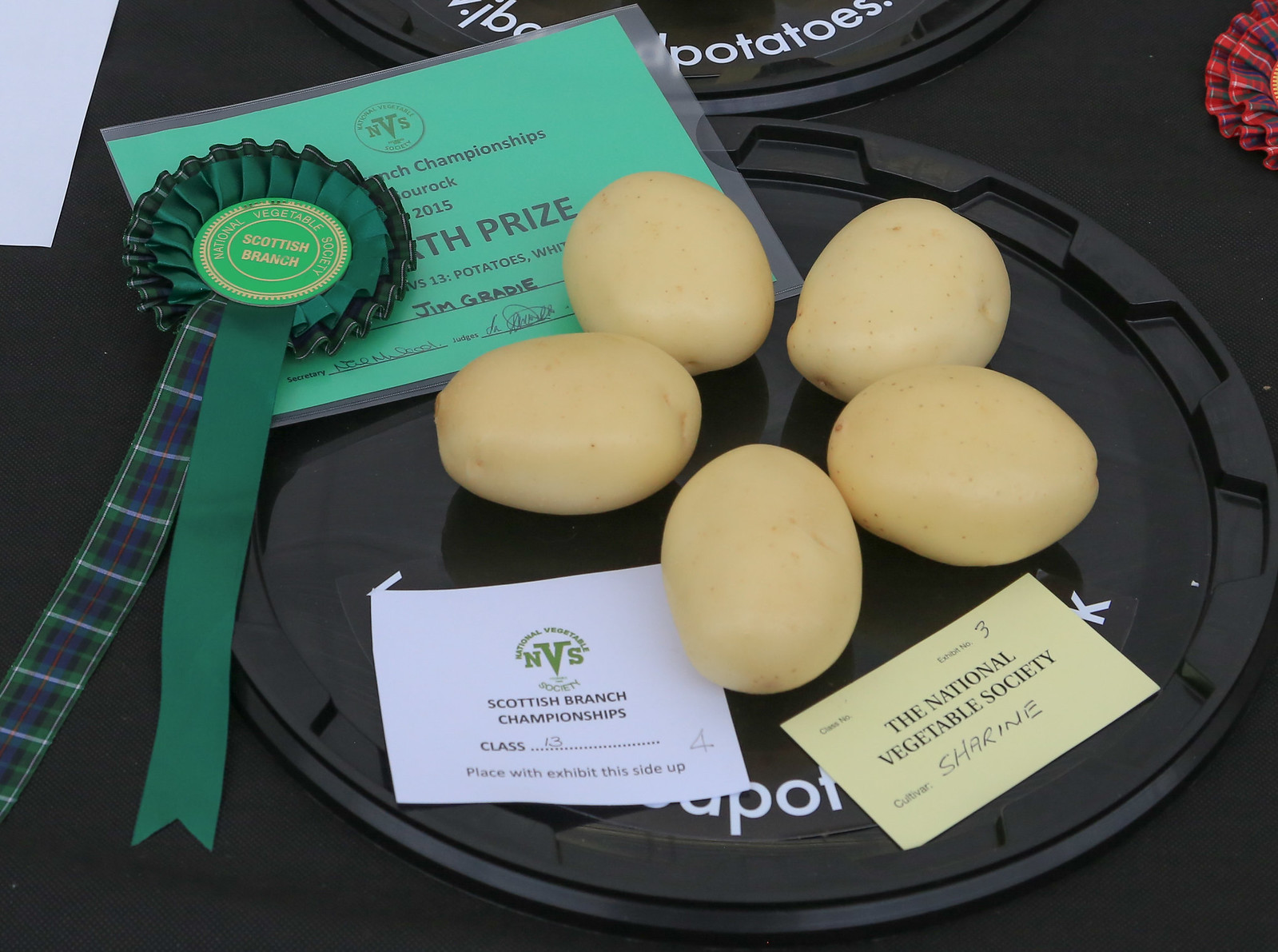In this image, a black disc-shaped plate with decorative edges is prominently featured, displaying five smooth, light tan potatoes arranged in a circular, almost flower-like pattern. The scene appears to be set on a table covered with black cloth. Surrounding the plate and potatoes are several notable items pertaining to an award.

In the top right corner of the image, a part of a red ribbon is visible. In the upper left corner, there is a piece of white paper detailing the competition's logistics. Above the plate, to the left, hangs a green ribbon with gold writing and designs, and a blue stripe down the middle, indicating it is from the Scottish Branch of the National Vegetable Society. This ribbon, partially obscuring a light green laminated paper, mentions a prize possibly for "sixth place" and the name "Jim Grady."

Additionally, on the bottom right of the plate, a label reads "National Vegetable Society" along with the word "Cultivar" and the name "Shereen." Another white card on the left side mentions "Class 13," directing the exhibit's placement and identifying the competition as part of the Scottish Branch championships. This card also suggests the exhibit was placed in fourth position, as implied by partial text on a green card. The entire display captures the essence of an agricultural competition, showcasing the careful presentation of these seemingly award-winning potatoes.